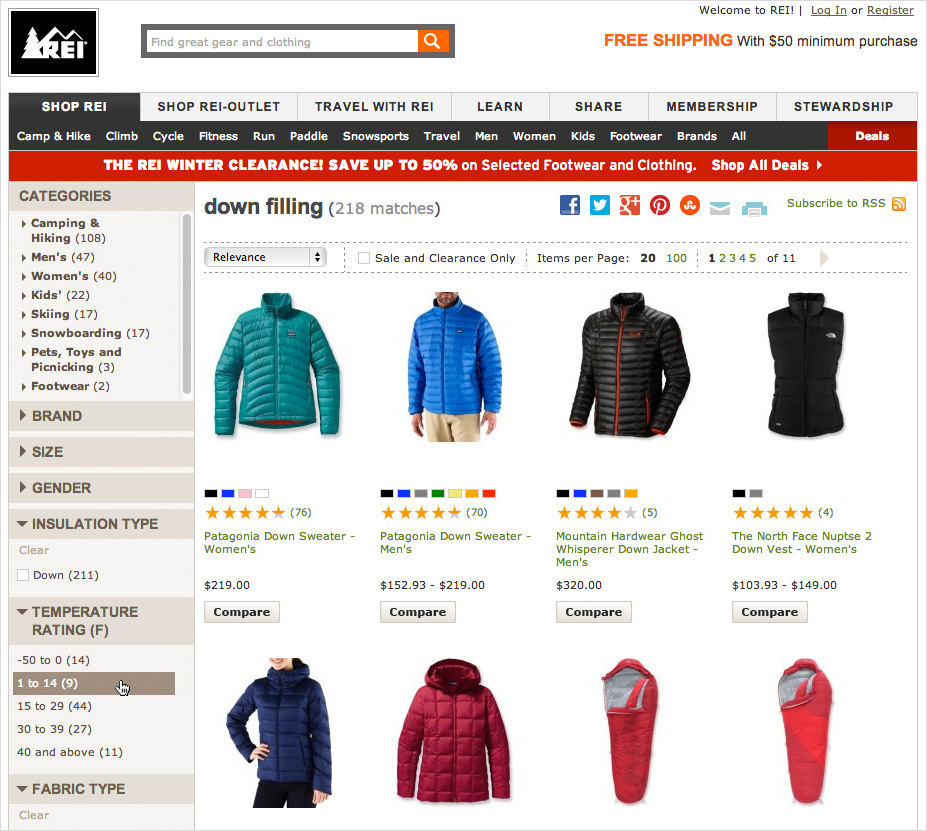The REI website appears to be dedicated to outdoor clothing and gear. In the top left corner, the logo consists of a black rectangle featuring a white silhouette of a pine tree with white mountains in the background. The bold, capitalized letters "REI" are displayed in white. Next to the logo, there is a search bar that includes a magnifying glass icon set against an orange square. Moving rightward, the phrase "FREE SHIPPING" is highlighted in bold, capitalized orange letters, followed by a smaller black text that states "with $50 minimum purchase."

A menu bar below the logo provides various navigation options. The "Shop REI" tab is currently selected, denoted by its dark gray background. The subsequent submenu lists categories such as Camp and Hike, Climb, Cycle, Fitness, Run, Paddle, Snow Sports, Travel, Men, Women, Kids, Footwear, Brands, and All. To the right of these selections, a red section with white lettering says "Deals."

To the right of the main menu, additional options include "Shop REI-Outlet," "Travel with REI," "Learn," "Share," "Membership," and "Stewardship," all displayed against a light gray background with black text.

On the left-hand side of the page, a beige rectangular area introduces the "Categories" section, marked by bold, brown, capitalized letters. Listed beneath are the categories: Camping and Hiking, Men, Women, Kids, Skiing, Snowboarding, Pets, Toys, Picnic, and Footwear. Each category features a dropdown menu for more specific options.